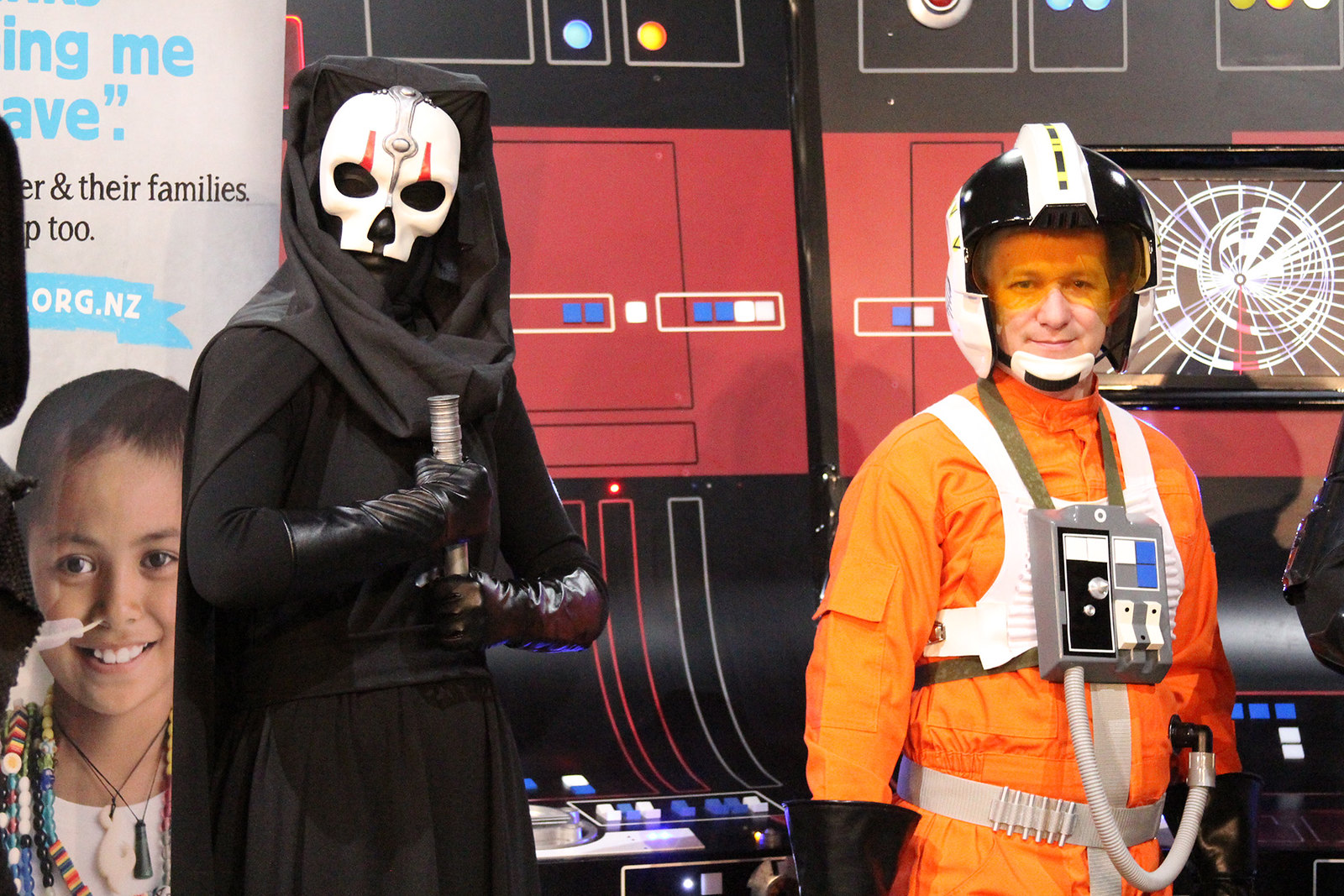In this vibrant and somewhat eerie photograph, taken possibly at a costume party or comic book convention, two individuals are meticulously dressed in elaborate Star Wars-themed cosplay. On the left, a figure cloaked entirely in black wears a hooded robe and a haunting skull-like mask adorned with black features and white trim, accentuated by striking red vertical lines over the eyes. Black gloves cover their hands, and they clutch what appears to be the base of a lightsaber or a metallic pipe-like object. To the right stands another character in a detailed pilot suit, featuring a predominantly orange jumpsuit paired with a white vest and a helmet with an orange-tinted visor, reminiscent of an X-Wing pilot from the Star Wars universe. This ensemble includes a silver, gray contraption with buttons and knobs, and hoses connecting back to the suit. This person directly faces the camera, unlike their masked counterpart. In the background, a faux futuristic cockpit filled with blue, white, red, and black buttons and knobs enhances the sci-fi atmosphere, along with a partially visible gray banner featuring an indistinct blue and black text, and a smiling child. The child, possibly in a hospital setting due to a noticeable nasal tube, has short brown hair and wears several necklaces, adding a touch of humanity amidst the otherworldly scene.